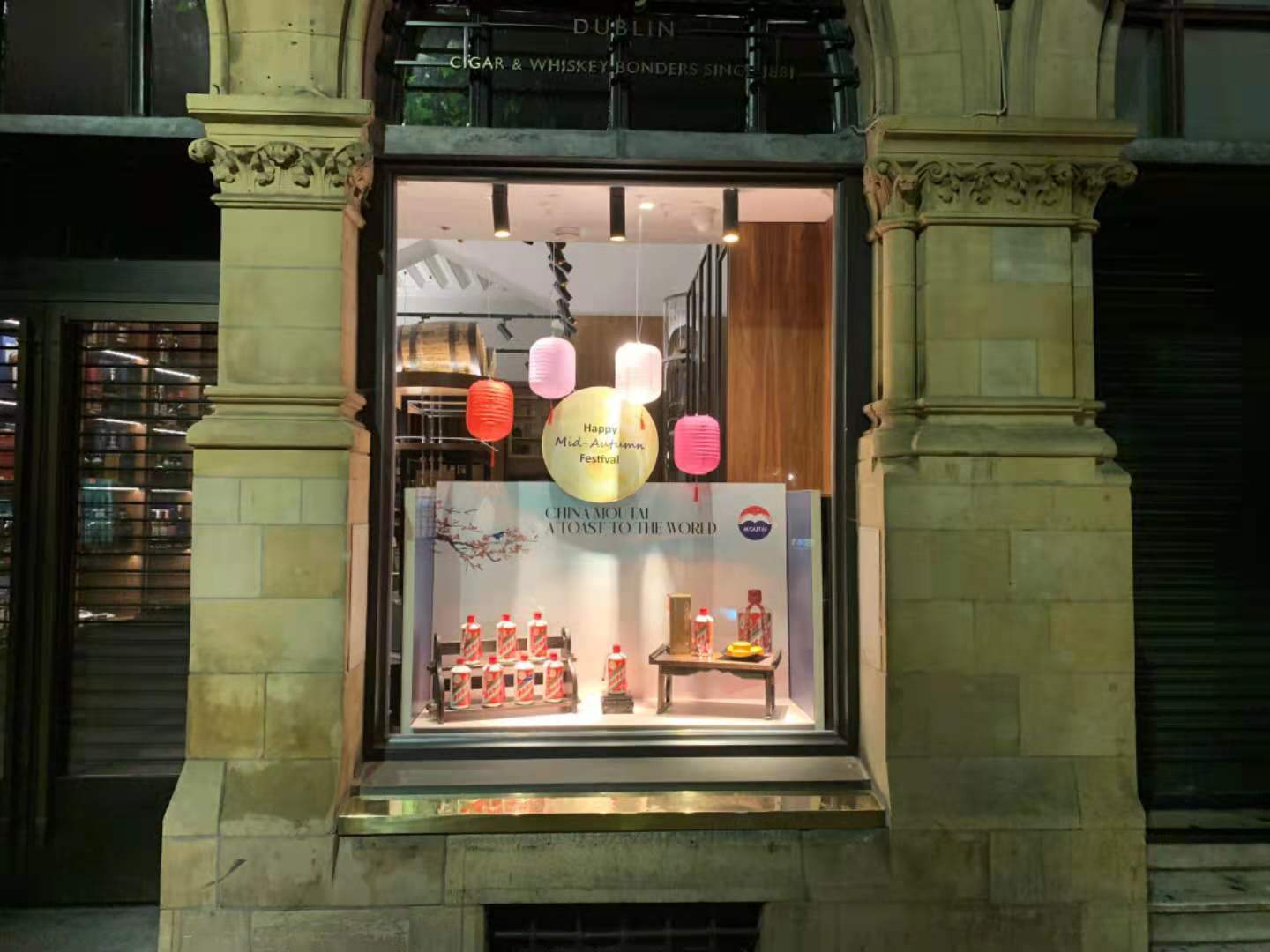This nighttime color photograph captures an intriguing storefront illuminated by hanging lights wrapped in vibrant, multi-colored material. Framed by distinctive light brown, almost yellowish, Gothic-style brick pillars adorned with intricate top decorations, the centerpiece is a large, black metal-framed picture window. This window features an enchanting display centered around the Happy Mid-Autumn Festival. The display includes a small shelf on the left holding seven spray-can-like items, a podium in the middle with a spray can on it, and a mini table on the right with another spray can and some hard-to-distinguish miscellaneous items. Above this arrangement, festive red, pink, and white paper lanterns hang, enhancing the celebratory ambiance. In the partially visible store behind, glass doors are seen to the left. The storefront proudly bears a sign above the arching window frame that announces "Dublin Cigar and Whiskey Bonder," adding to its unique and historic charm. Additionally, the display backdrop features black text, stating, "China, a toast to the world," adding an international festive flair.